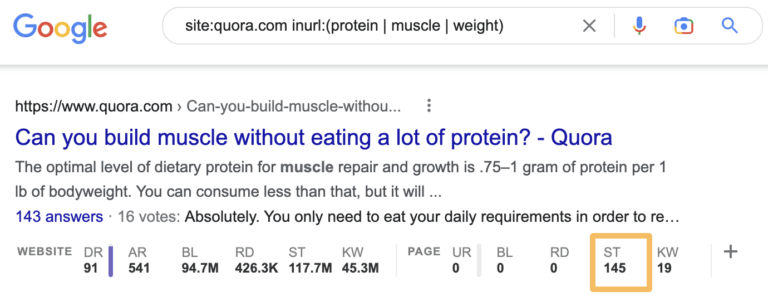A Google search for "protein and muscle weight" is displayed on the screen. At the top left corner, the iconic Google logo is visible with its distinctive colors: uppercase blue G, lowercase red O, lowercase yellow O, lowercase blue G, lowercase green L, and lowercase red E. The search query utilizes advanced functions, specifying results from Quora with the command "site:quora.com" and narrowing the search using "inurl", followed by the keywords "protein", "muscle", and "weight" separated by dividers.

Next to the search bar, the clear (X) button is present, followed by a blue microphone icon, with its base colored red. There is also a multi-colored (blue, red, green, and yellow) camera symbol for image searches and a blue magnifying glass indicating the search button.

The top search result from Quora.com is highlighted in blue and reads, "Can you build muscle without eating a lot of protein?" Below, a snippet provides a brief answer: "The optimal level of dietary protein for muscle repair and growth is 0.75 to 1 gram of protein per one pound of body weight. You can consume less than that, but it will..." The rest of the text is cut off. Additional search stats are partially visible underneath the description.